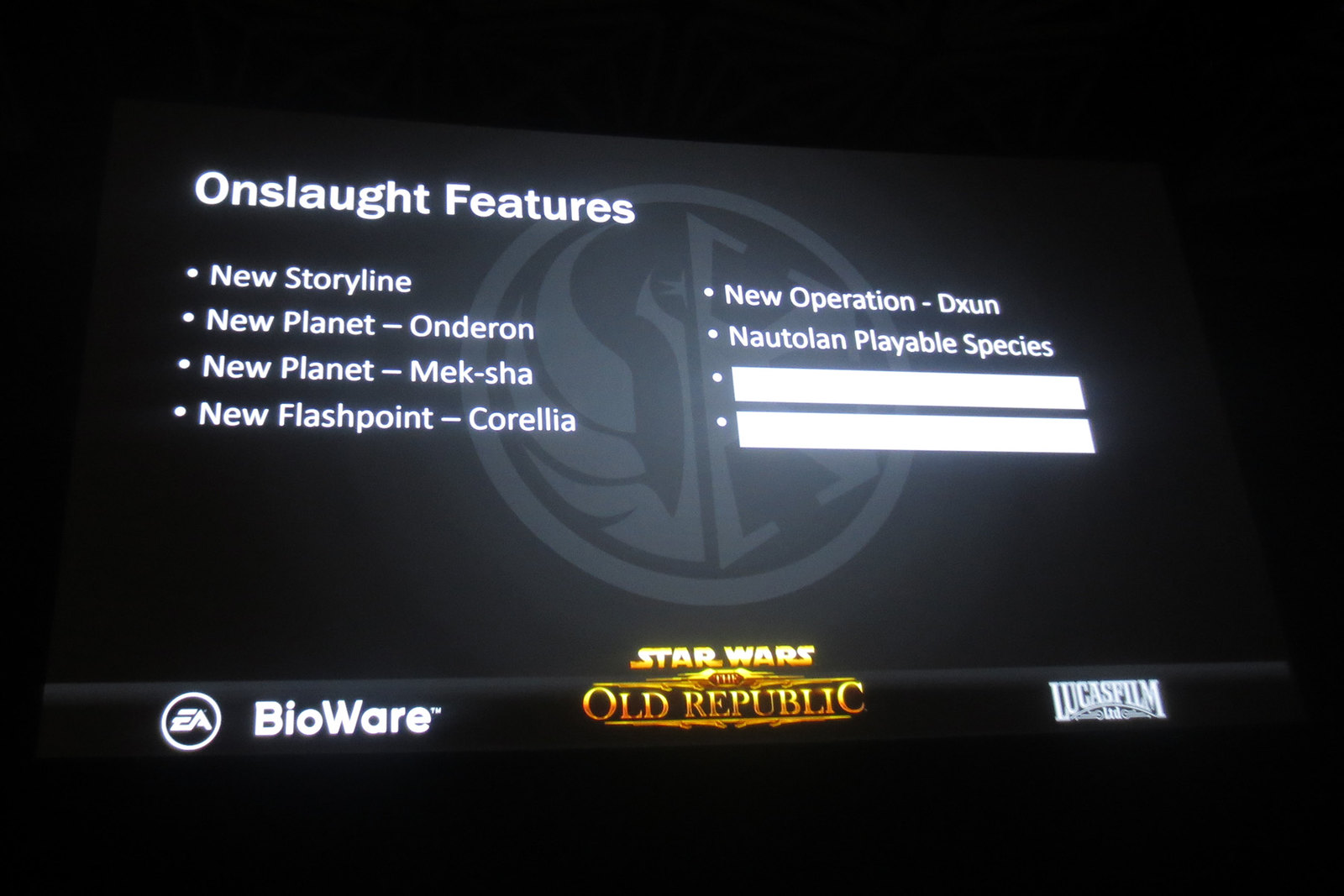The image is a screenshot of a computer or television screen, prominently displaying information about "Star Wars: The Old Republic." The background is predominantly black, with a faint, gray, hemispherical emblem in the center. In the bottom center, the title "Star Wars: The Old Republic" is written in gold, accompanied by logos for EA, BioWare, and Lucasfilm on either side. Above the title, at the top center, white text is divided into two columns under the heading "Onslaught Features." 

The left column lists:
- New Storyline
- New Planet: Onderon
- New Planet: Meksha
- New Flashpoint: Corellia

The right column lists:
- New Operation: DXUN
- Nautolan Playable Species

Additionally, two empty rectangular boxes are present, seemingly meant for user input or additional information. The image is entirely against a black background, with the mentioned text and logos being clearly visible in their respective positions.